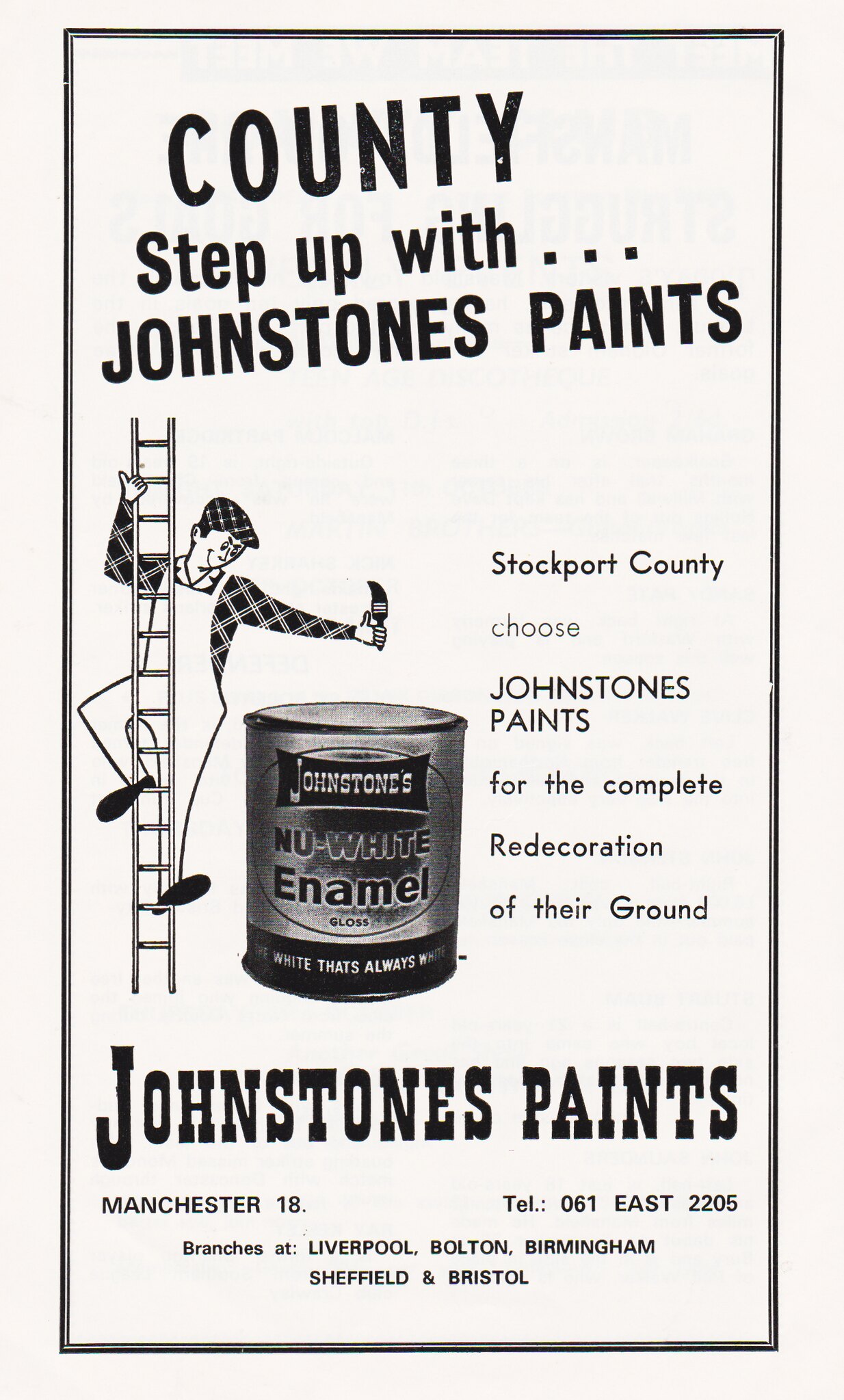This vintage advertisement for Johnstone's Paints highlights Stockport County's choice for their complete ground redecoration. The ad is black and white, with bold, capitalized text at the top that reads, "COUNTY, Step Up with Johnstone's Paints." A cartoon man, dressed in a matching plaid beret and shirt under white overalls, is shown climbing a ladder. He holds a paintbrush in his left hand and looks down toward a gallon can of Johnstone's New White Enamel Gloss paint, labeled "The white that's always white." The center of the ad features this paint can prominently. To the right of the can, the ad reiterates the theme: "Stockport County chooses Johnstone's Paint for the complete redecoration of their ground." Contact information is displayed at the bottom, listing the Manchester headquarters with telephone number 061 East 2205, along with branches in Liverpool, Bolton, Birmingham, Sheffield, and Bristol.